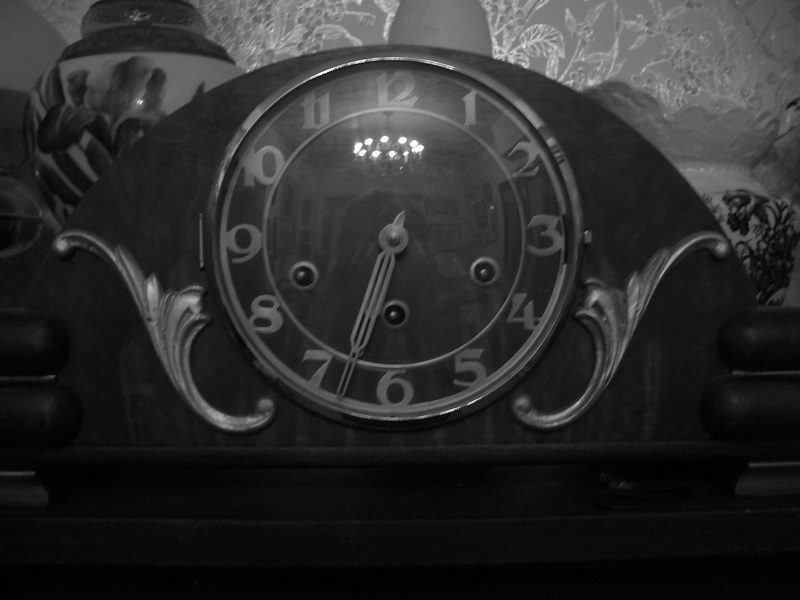The image showcases a large, black and white vintage desk clock with a distinct antique charm. The clock, which appears to have a wooden body with a horizontal rectangular base and a rounded top, is situated on a dark surface, possibly a mantel or nightstand, suggesting it is in a homely, likely living room, setting. The face of the clock is round with large, clear numerals from 1 to 12, and the hands are pointed together slightly to the left, indicating a time around 25 minutes to 7. 

Distinctive decorative detailing is present around the clock. Notably, the sides feature embellishments resembling a backward "S" shape with wing-like extensions toward the center, possibly made of pewter. There are three centered dots on the clock face, which might be part of a chiming mechanism or for another function. 

The background of the image includes textured wallpaper or curtains and a large vase adorned with floral patterns. Another smaller vase or potentially a plant can be seen to the right, adding to the vintage aesthetic of the setting. A noticeable reflection of light is visible on the glass covering the clock face, which may have a mechanism to open it for maintenance. This detailed scene is captured in a nostalgic black and white photograph, enhancing the timeless quality of the antique clock and its surroundings.